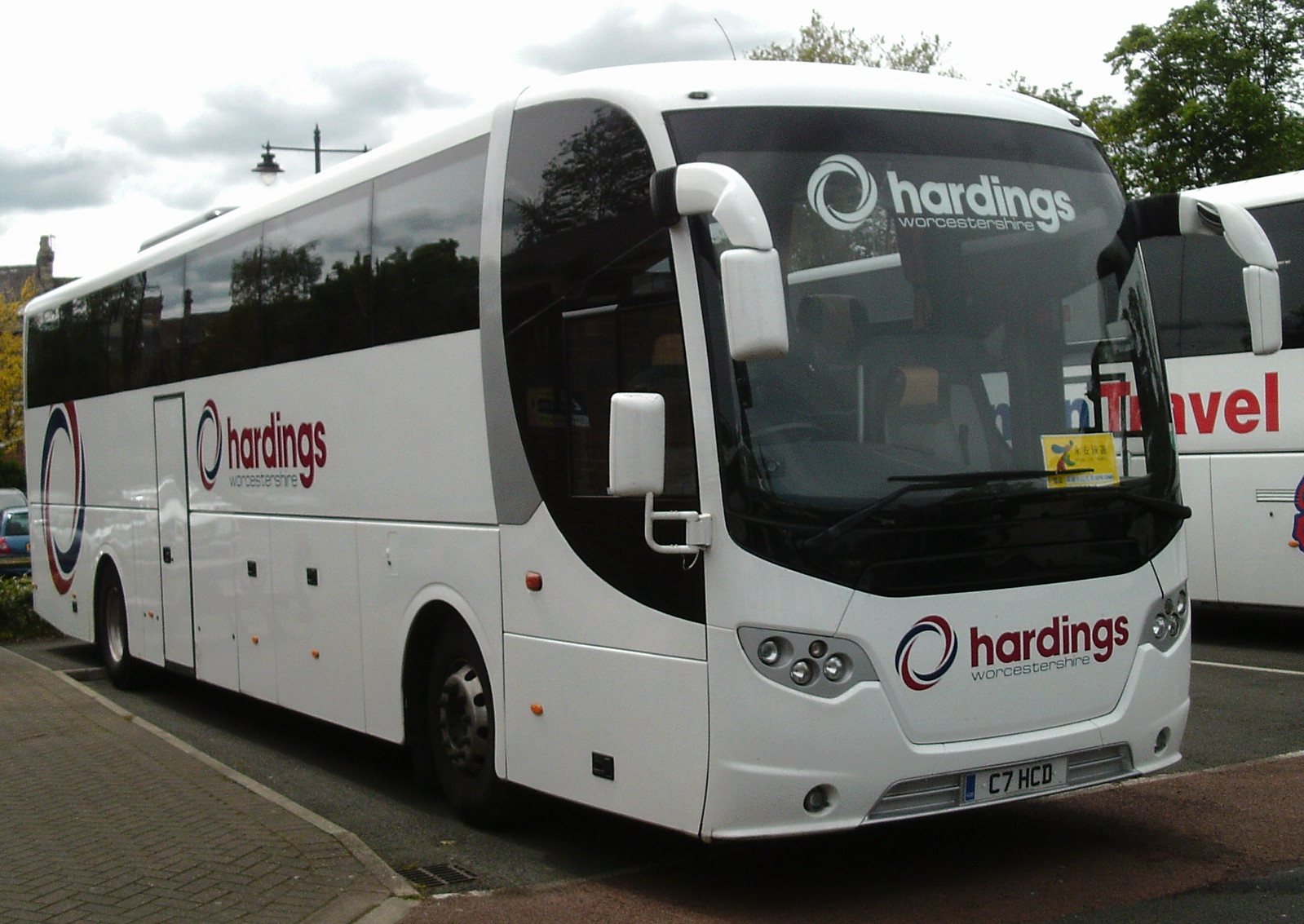The photograph depicts a Harding's Worcestershire tourism bus parked in a lot with another white travel bus stationed next to it on the right. The main bus prominently displays a circular spiral logo and the word "Harding's" on both the front and side, with "Worcestershire" written beneath. It has a sleek, curved windshield, small modern headlights, and the license number C7HCD. The bus features dark tinted windows and side mirrors that confer a bug-like appearance with their angled positions. The buses are parked on pavement, bordered by a reddish brick sidewalk with a cement curb. The backdrop includes overcast skies and some trees, with hints of urban elements like a city light fixture and a distant building chimney amidst the foliage. No people are visible in the image. The image dimensions are 8 inches wide by 7 inches tall.